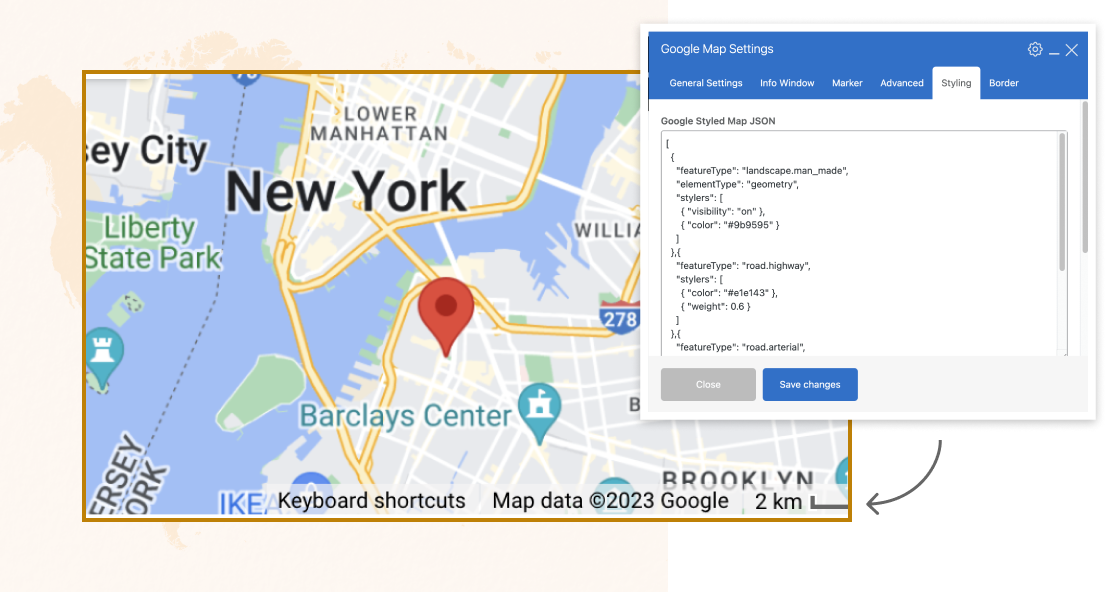The image showcases a detailed view of a pop-up menu positioned on the top right corner of a screen, labeled "Cookie Map Settings." The menu contains several tabs, including "General Settings," "Info Window," "Maker," "Advanced," "Styling," and "Bot," with the "Styling" tab highlighted in white text on a black background, while the other tabs have white text on a blue background. 

Below the tabs, there is a section displaying a JSON code editor for "Cookie Style Map," where the code is written in black text against a white background. The code specifies various styling parameters such as "landscape," "geometry," "visibility," "color," "feature type styles," and "weight."

At the bottom of the menu, two buttons are present: a gray "Close" button and a blue "Save Changes" button. Additionally, there is an arrow pointing to the left, indicating a return to the main page being edited.

On the left side of the image, there is a map of New York. The map uses distinct colors to differentiate various elements: blue for sea areas, green for parks and vegetation, gray for land, white for minor roads, and yellow for main roads. At the bottom of the screen, it includes information about "Keyboard Shortcuts," "Map Data," and references "2023 Cookie."